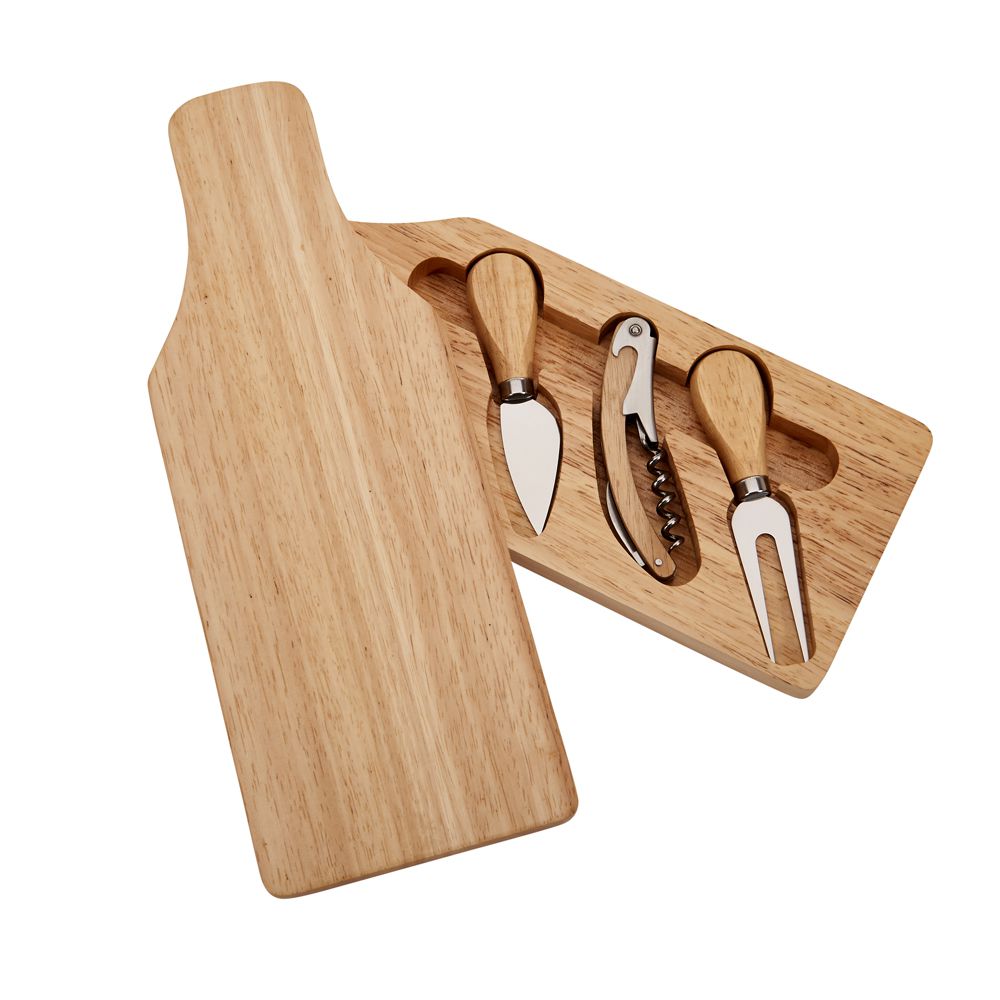This image presents a sophisticated, two-tiered wooden cheese board designed for entertaining. The top portion, resembling a bottle shape with a wider neck that curves gracefully upward, slides open to reveal an organized interior storage compartment. Inside, the recessed compartment houses a selection of tools, including a corkscrew for wine bottles, a short-handled cheese knife for spreading or cutting, and a double-pronged fork potentially used for grabbing meats. All tools feature wooden handles that match the board's natural wood grain aesthetic. The photo is taken from above, showcasing the full layout of the board against a minimalist white background, emphasizing the board's functionality and sleek design.